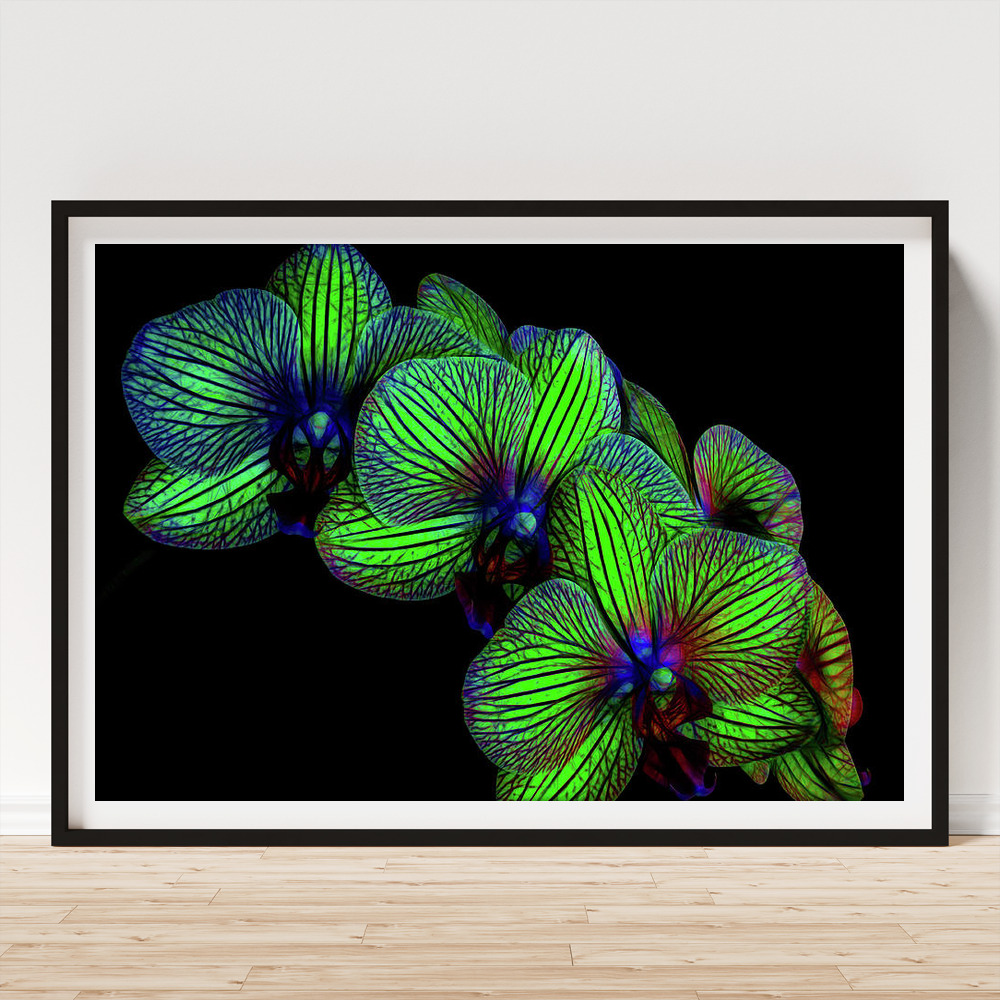The image depicts a large rectangular picture frame leaning against a light wood-tiled floor beneath a grayish-white wall with a white baseboard on either side. The frame itself is thin and black, with a white inner border surrounding a solid black background. Central to the picture are three prominent flowers with lime or neon green petals. The petals feature intricate purple, reddish, and blue veins, adding a vibrant contrast. The center of each flower has green buds mingled with bluish-purple and reddish hues. The overall composition and the wooden floor suggest that it might be a computerized image, and there are no identifying details about the artist or the origin of the picture.